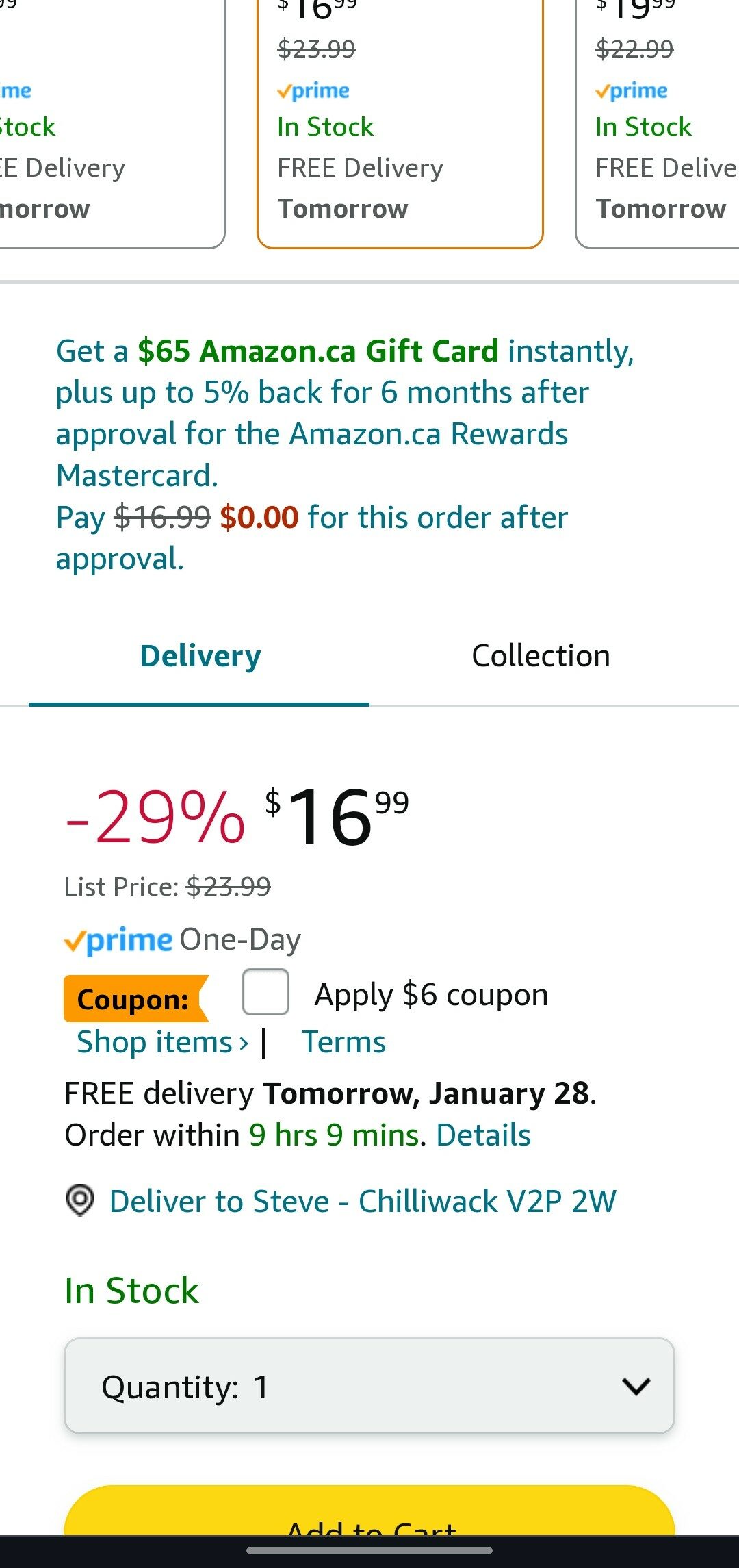The image appears to be a screenshot of an Amazon product page on a mobile device, but various elements are cut off or obscured by borders. Here's a detailed description of the content visible in the image:

At the top, the typical information such as the time and battery charge is missing. The product the person is interested in buying is not clearly visible. The prices seem to vary by size, but some details are obscured by a gray border.

Visible text includes the word "Delivery," while the rest is cut off. A box with a brown background shows a price of $16.99, reduced from $23.99, which is crossed out. Below this, in blue text, it says "Prime," and underneath that in green text, it states "In Stock." Below in black text, it mentions "Free delivery tomorrow."

Another gray box shows a price of $19.99, reduced from $22.99, which is also crossed out. Next to the blue word "Prime," there is an orange checkmark. In green text, it says "In Stock," followed by "Free delivery tomorrow," though part of the word "delivery" is cut off.

A gray line runs horizontally across the image. Below, in teal text, it mentions getting a $65 Amazon.ca gift card instantly, plus up to 5% back for six months after approval for the American.ca Rewards MasterCard, with details about Amazon Pay.

There is a mention of a price being reduced from $16.99 to $0.00 in red, indicating a special offer after approval for the card.

The overall image gives an impression of an Amazon product listing with multiple price offers and delivery options, some of which are partially cut off by borders.